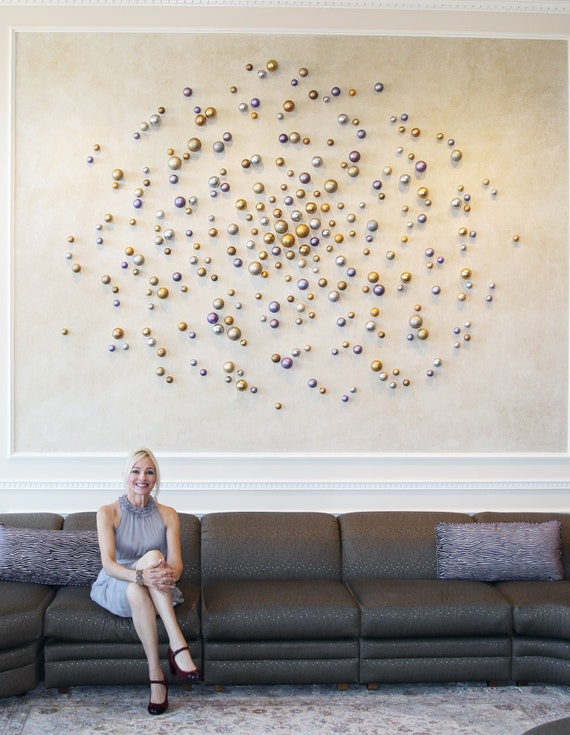In this photograph, a smiling blonde woman is seated on the lower left side of a wide, dark gray leather couch that stretches across the frame. She is wearing a sleeveless light gray dress along with black high heels, and her legs are elegantly crossed with her hands clasped over her knee. The setting looks like a lobby area, possibly in a hotel, and the couch has sectional seating divided by rectangular-shaped throw pillows placed at either end of the couch.

The background is dominated by a large, eye-catching art piece mounted on the wall. This artwork features a mesmerizing array of orbs in various colors including gold, silver, chrome, brass, purple, lavender, and shades of blue and gray. These orbs are tightly clustered towards the center and radiate outward in a swirly, spiral, almost random pattern, all framed by a white border. The comprehensive scene blends the woman's poised grace with the dynamic and colorful backdrop, creating a striking visual composition.